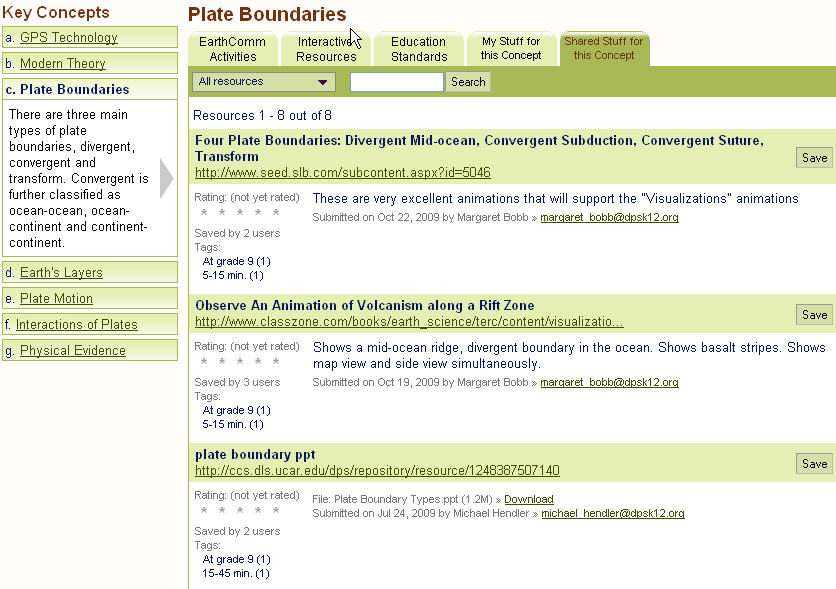**Caption:**

The landing page design features a mix of white, light green, and dark green hues with gray and green text on a white background, creating a clean and organized look. There is no border around the image. 

At the very top, "Plate Boundaries" is prominently displayed in bold, dark brown text. Beneath this title, a series of light gray tabs stretch horizontally across the screen. The tabs read: "Earth Calm Activities" and "Interactive Resources" with brown text, followed by "Education Standards," "My Stuff for This Concept," and a highlighted tab labeled "Shared Stuff for This Concept" in dark green.

A dark green ribbon runs across the screen below the tabs, containing the text "All Resources" inside a light gray box with a dropdown arrow, positioned next to a white search bar on the right.

On the main section of the page, a white background hosts "Resources 1-8 out of 8" in navy blue text. Below this, a light green ribbon features a list of four plate boundary types in navy blue text: "Divergent Mid-Ocean," "Convergent Subduction," "Convergent Suture," and "Transform." 

Underneath these headings, a link to a webpage is presented in green text, followed by a white ribbon that contains the phrase "These are very excellent animations that will support the visualizations animations" in navy blue text. This is further detailed with submission information stating, "Submitted on October 22, 2009 by Margaret Bob," accompanied by her email address in gray text. The page has a busy layout with a blend of various text colors and sections, designed to offer a comprehensive range of information at a glance.